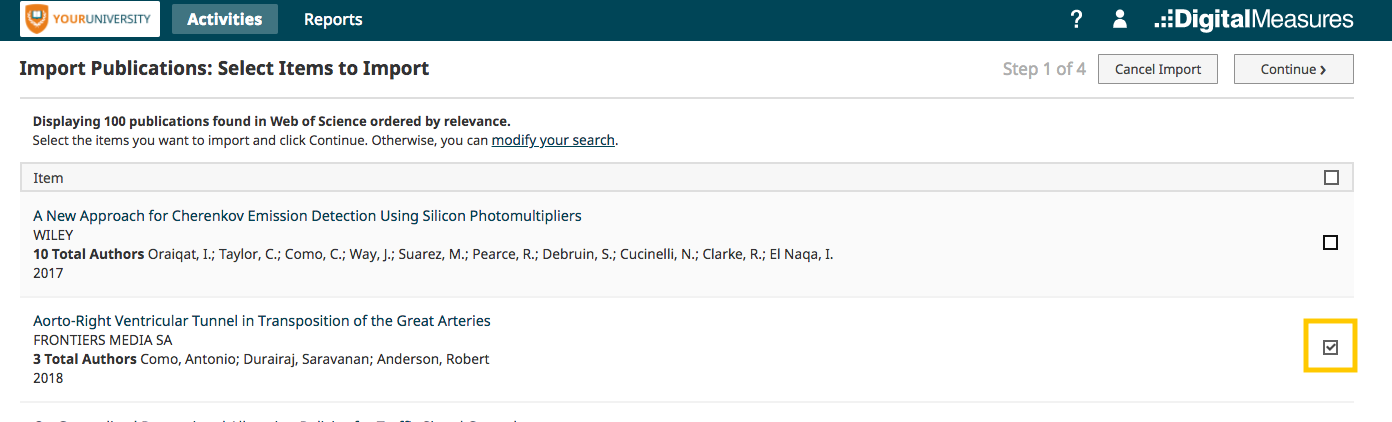The image is a screenshot from the "Your University" website, prominently displayed at the top of the page. The interface showcases various tabs, including "Activities" and "Reports," with the "Activities" tab currently highlighted. On the far right, there is a label titled "Digital Measures," which might refer to a publication or company. Next to it are icons for user settings and help, represented by a user profile and a question mark icon, respectively.

The central part of the interface is titled "Import Publications: Select Items to Import." It indicates that there are 100 publications found in Web of Science, listed by relevance. However, the visible section of the screenshot only displays two of these publications. Among these, the second publication is selected, highlighted with a checkbox on its right side and outlined in yellow, drawing attention to this selection action.